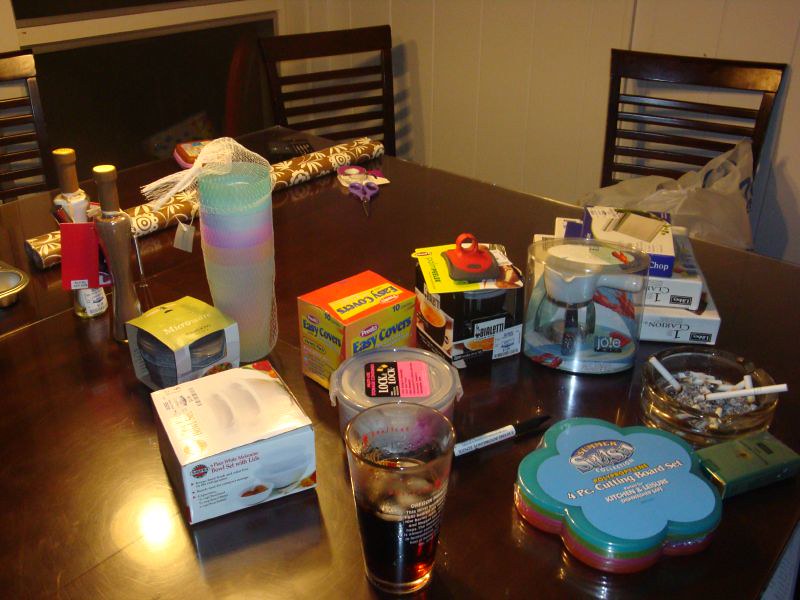In this vibrant color image, a cluttered table is brimming with an array of items. Dominating the scene is a whimsical four-piece cutting board set designed in the shape of flowers. To the right, a cup filled with ice and Coca-Cola adds a refreshing touch. Nearby, a clear, circular ashtray holds several used cigarettes, adjacent to a green cigarette pack. A neatly stacked assortment of plastic cups sits in a container, adding to the disarray. A visible box labeled "Easy Covers" hints at kitchen accessories. In the top left corner, a pair of purple scissors rests next to a roll of brown patterned wrapping paper, with a pack of Scotch tape partially hidden behind them. The brown chairs surrounding the table cast distinct shadows on the white wall, enhancing the sense of depth in the composition.